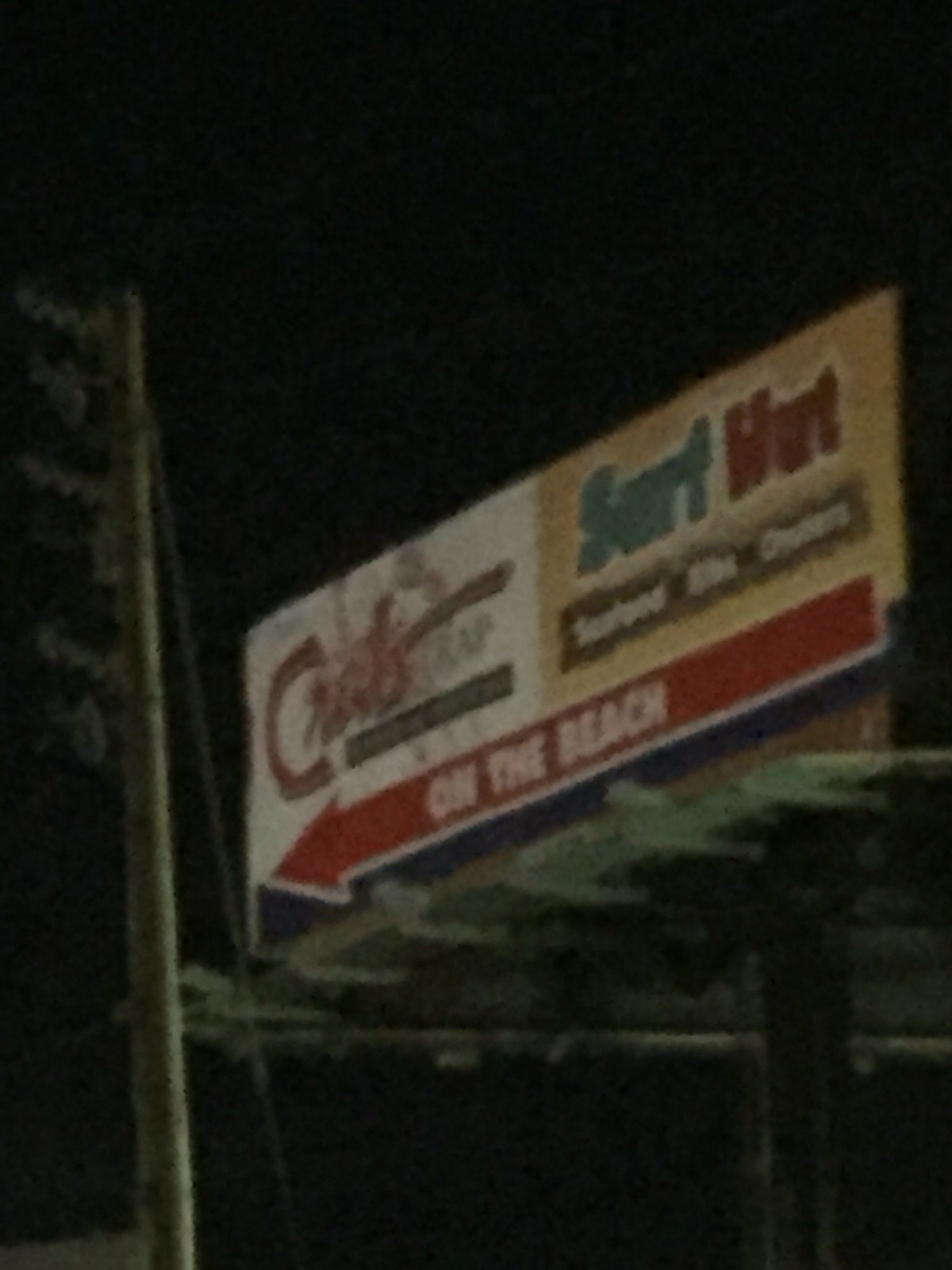This color photograph, taken at night, showcases a dark and blurry snapshot of a horizontal billboard, apparently located at the beach, mounted on a metal scaffolding structure. The sign is divided into two distinct sections: the left half features a white background with mostly illegible brown and red text, including the word "Crab" in red, and a worn-off logo. The right half has a tan or beige background displaying "Surf" in green and "Hut" in red. Below this text, on the right side, is another black rectangle with some unreadable white text. Below the entire sign, stretching across both sections, is a thick red arrow pointing to the left with the phrase “On the Beach” prominently displayed in large white block letters. The billboard is illuminated by front lights, casting shadows on the dark metallic scaffolding and highlighting a vertical pole that runs up the left side of the image.